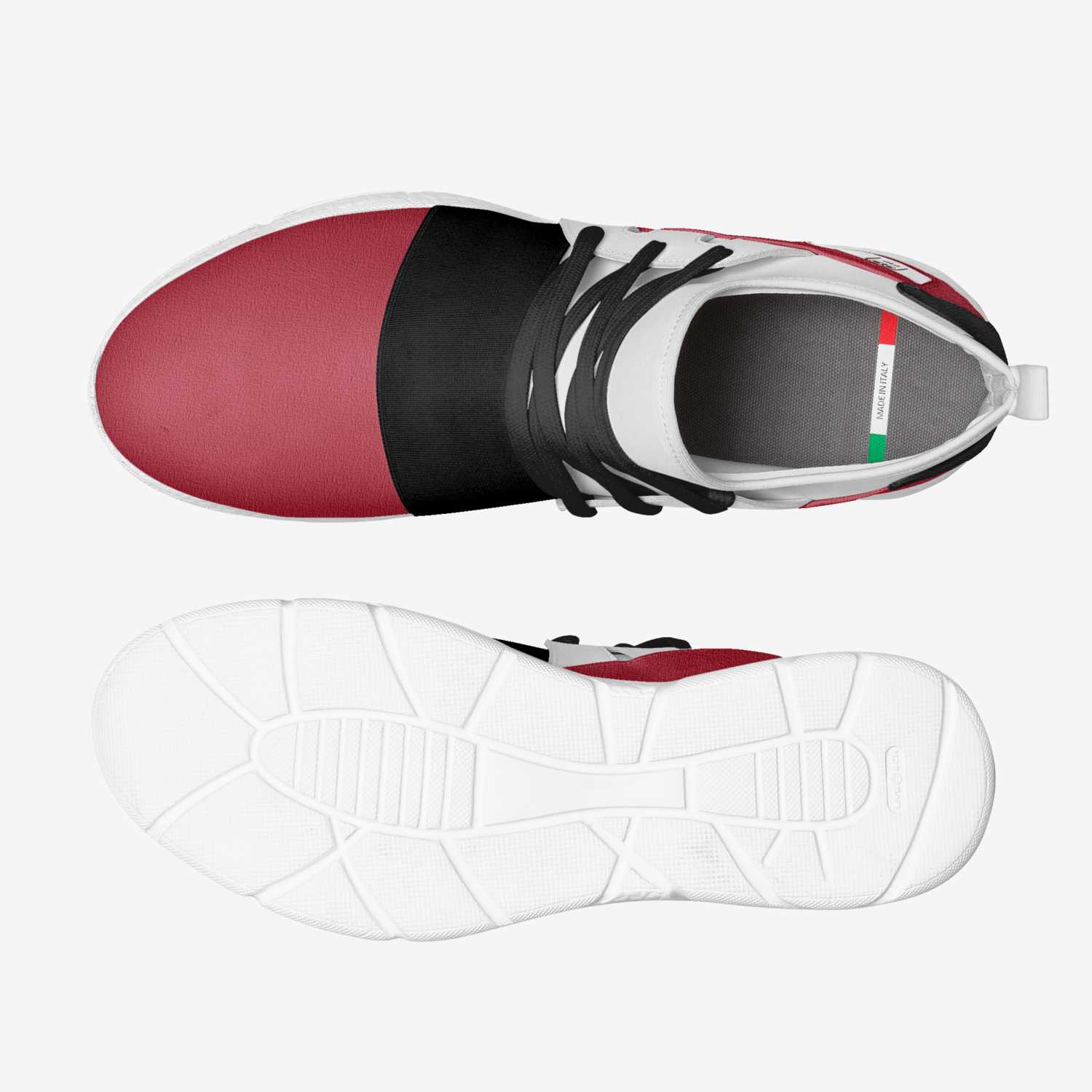The image showcases a pair of shoes meticulously placed on an all-white background. The left shoe is upright, providing a top view that reveals a versatile design of raspberry red at the top, transitioning into a black mid-section, and culminating in a clean, bright white at the toe area. The shoe features black laces and a gray insole speckled with white and gray dots. A vibrant tag inside the heel, bearing green, white, and saffron stripes, denotes its Italian craftsmanship. The right shoe is inverted to expose its sole, which is bright white with intricate lines forming a striking pattern. This detailed arrangement, set against a minimalist white background, highlights the shoes' modern aesthetic and high-quality craftsmanship.